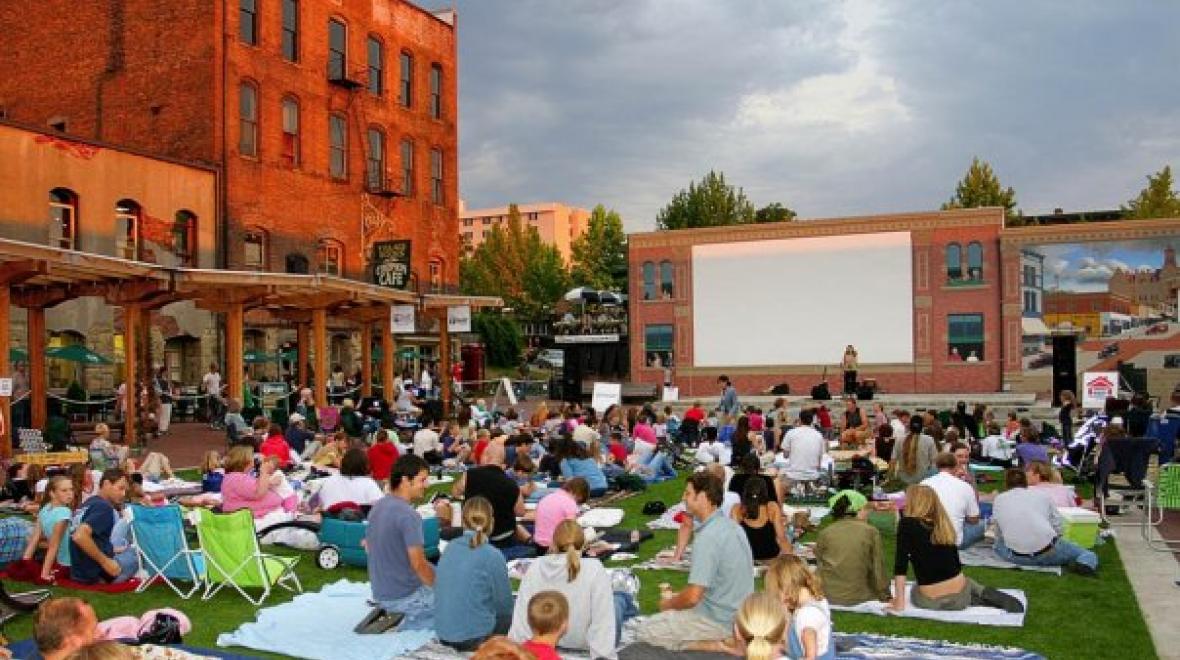This detailed scene captures an outdoor movie gathering in a grassy courtyard nestled between several brick buildings. On the left stands a vintage, red brick, four-story building with ground-floor shops and a sidewalk flanked by a concrete awning supported by pillars. Facing this building is a two-story brick structure with a large white movie screen, ready for an upcoming film screening. Adjacent to this is another brick building adorned with a city-themed mural, while a larger brick building peeks through the trees in the distance.

In the foreground, approximately a hundred people, predominantly young, are seated on various blankets, towels, and a few folding chairs in green and blue. They sit cross-legged, eagerly awaiting the movie to start. The atmosphere is vibrant with people wearing colorful clothing—reds, blues, whites, greens, and pinks—against the backdrop of manicured, lush green grass.

The sky is gray and overcast, yet the scene is warmly lit by the orange hues of the setting sun visible across the buildings. It’s a lively and inviting moment, full of anticipation, as daylight begins to fade, setting the stage for a communal cinematic experience.